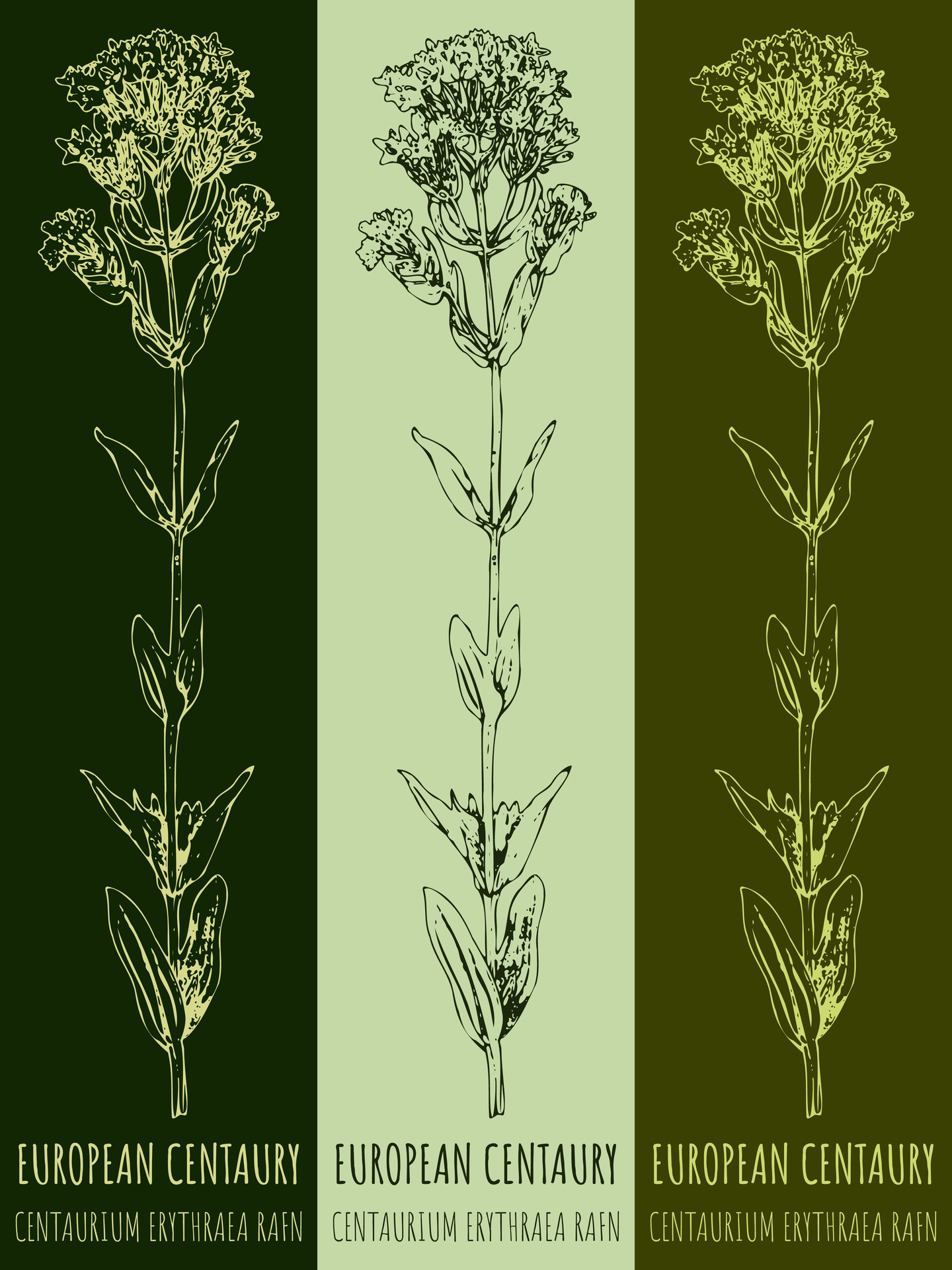The image is a detailed poster showcasing three vertically oriented panels side by side. Each panel features an identical depiction of a tall, elegant plant with a long stalk adorned by symmetrical sets of leaves and culminating in a cluster of flower buds. The background colors of these panels vary from left to right: the leftmost is a very dark green, the center is a very light green, and the rightmost is a medium shade of green, darker than the center but lighter than the left panel. Each plant illustration is rendered in a gold color, prominently standing out against the different background hues. Below each panel, the text reads "European Centaury Centaurium Erythraea," indicating the plant species. This text is consistent across the three panels, highlighting a botanical or event-related theme centered around the European Centaury plant.